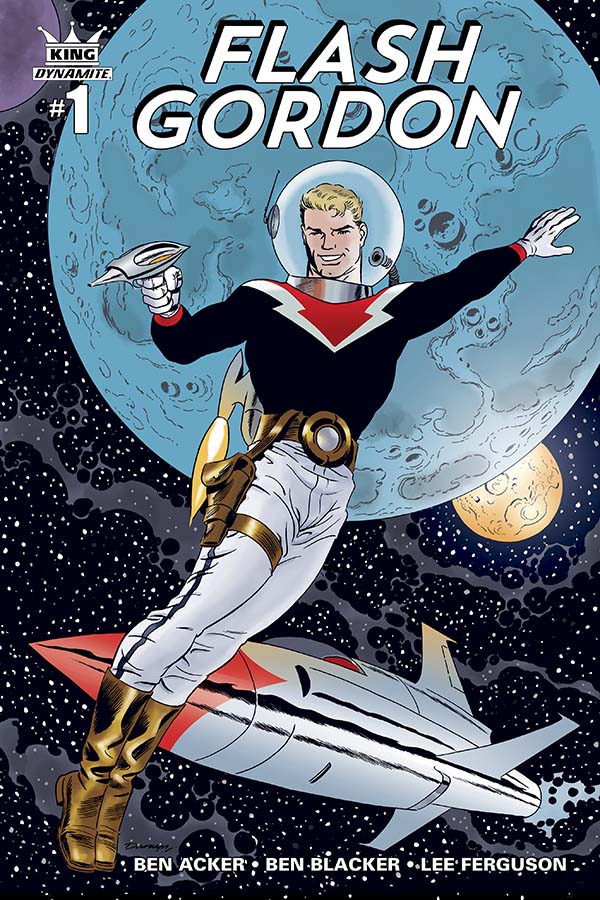The comic book cover depicts Flash Gordon from the 50s in a vibrant and detailed scene. At the very top, "Flash Gordon" is prominently displayed in bold, white capital letters with a black outline, against a large blue depiction of the world. In the upper left corner is a small white crown with the word "King" above "Dynamite" and a big number "1" in white, signifying the first issue.

Flash Gordon is positioned centrally, appearing to float in space with a space helmet on that resembles a fishbowl. His attire includes a black shirt adorned with a red arrow, topped with white detailing, white pants, gold boots, and a gold belt with a matching buckle. A silver ray gun is in his right hand, pointed forward, while his left hand extends upwards. His gold holster, attached to his leg, is designed to carry his gun. Behind him, a rocket ship with a silver body and red nose cone hovers in the background, alongside two celestial bodies that accentuate the space setting.

At the bottom of the cover, the names of the artists, Ben Acker, Ben Blacker, and Lee Ferguson, are displayed in bold white letters.